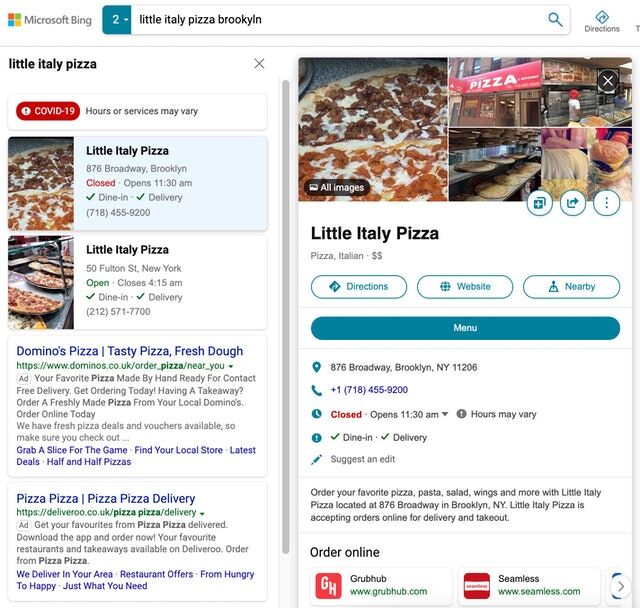A detailed caption for the described image could be:

"This is a screenshot of a Microsoft Bing search results page for 'Little Italy Pizza, Brooklyn.' The search bar at the top shows the number '2' with a dropdown arrow, accompanied by the search text 'Little Italy Pizza, Brooklyn.' Below, there is a 'Directions' tab.

On the right side, the main search result is highlighted in a red banner, indicating potential variations in hours of service due to COVID-19. The top listing is for 'Little Italy Pizza' located at 876 Broadway, Brooklyn, which is currently closed but will open at 11:30 AM. The listing includes options to check for dine-in and delivery services, along with a contact number, 718-455-9200.

Another listing shows 'Little Italy Pizza' at 50 Fulton Street, Brooklyn, New York, which is open until 4:15 AM. This listing also provides dine-in and delivery options, along with contact numbers, 212-571-7700.

Below these, there are additional listings for 'Domino's Pizza,' noted for its tasty pizza and fresh dough, and another pizza delivery service.

To the right of the listings is a photo gallery featuring images of Little Italy's pizzas, storefront, and kitchen. The section also includes details about the restaurant's Italian pizza offerings, its pricing category denoted by a dollar sign, and options to get directions, visit the website, and view the menu. The specific details like the address, phone number, and operating hours are reiterated, along with a promotional message encouraging customers to order their favorite dishes such as pizza, pasta, salad, and wings from 'Little Italy Pizza' located at 876 Broadway, Brooklyn, New York. The restaurant accepts online orders for delivery and takeout through services like Grubhub and Seamless, with a button provided to 'Order Online.'"